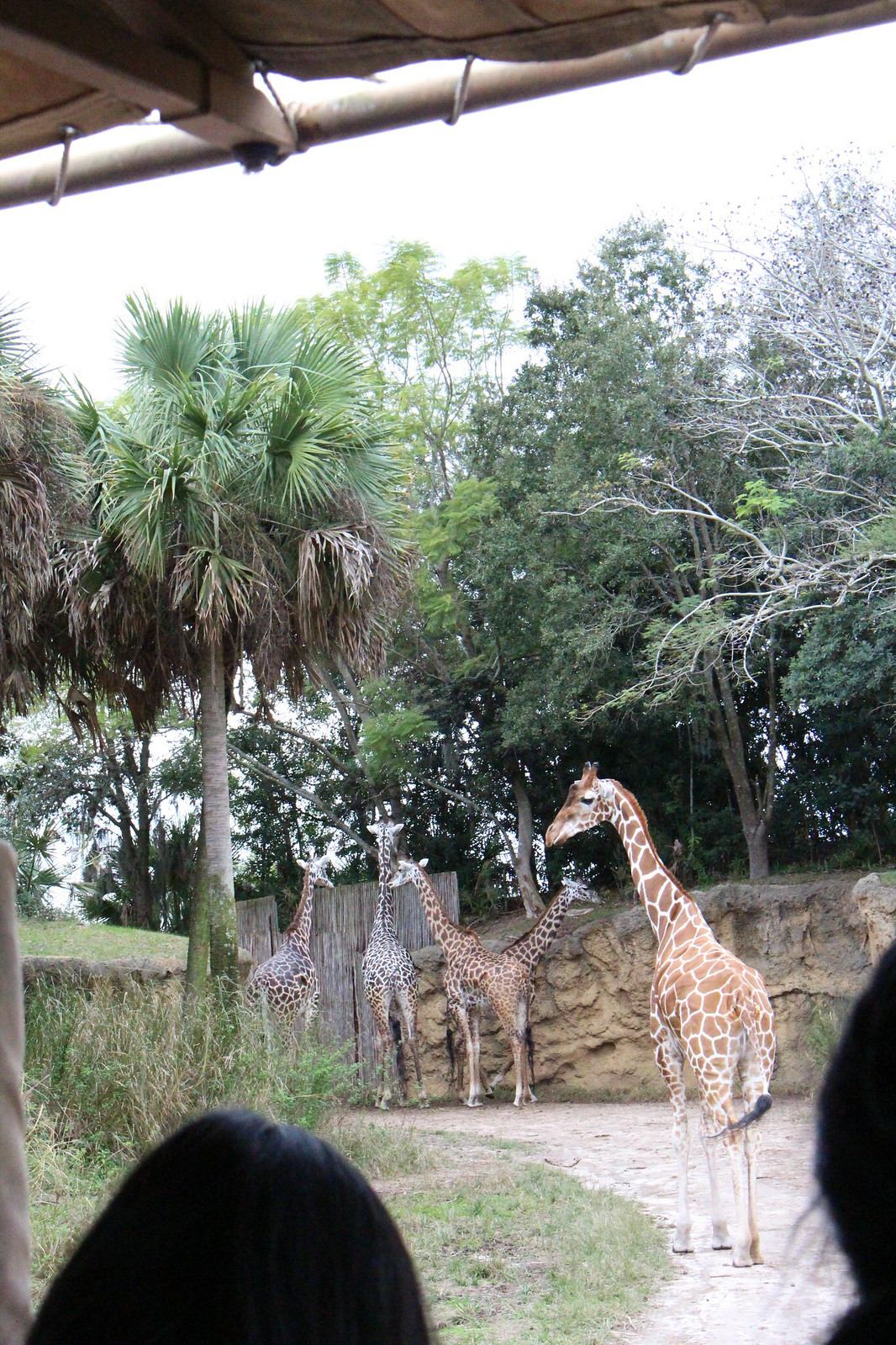The image captures a lively scene at a zoo or wildlife park, providing a rich view of giraffes in their enclosure. In the foreground, the backs of two people’s heads are visible, suggesting they are on an open-sided tour bus with a tarp roof. The closest giraffe to the camera, slightly younger and lanky with a traditional orange and brown pattern and a tuft of dark hair on its tail, stands with its body facing away but its neck turned to the left, gazing at something out of frame. Further back in the enclosure, four more giraffes are dispersed: a pair of taller giraffes in the far back, seemingly parental figures, with another facing away near a fence; and two smaller giraffes, one grazing and the other looking up at the taller ones. The giraffes are surrounded by a mixture of grass and worn, bare dirt. The enclosure is bordered by a tall wooden fence on the left and a stone wall enhanced with two palmetto trees. Mature trees, both tropical and deciduous, stand atop a hill behind the stone wall, providing a lush backdrop to the scene.